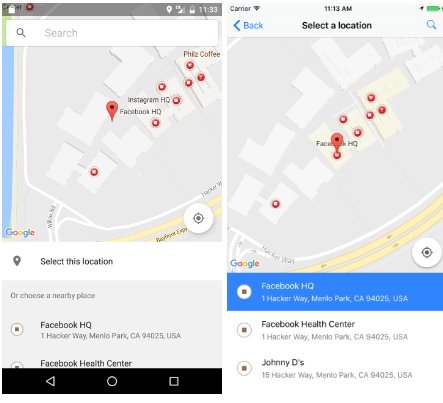Two phone screenshots display a map featuring notable locations near and around Facebook HQ. The first screenshot shows a general map interface, prompting the user to select or search a location. Several prominent landmarks are labeled, including "Facebook HQ," "Instagram HQ," and "Philz Coffee," among others. Text on the screen instructs the user to "Select this location or choose a nearby place," with Facebook HQ situated at 1 Hacker Way, Menlo Park, California, 94025 USA, also spotlighting the Facebook Health Center.

The second screenshot indicates that Facebook HQ has been selected as the specific location. Details include the address 1 Hacker Way, Menlo Park, California, 94025 USA. Beneath this, the Facebook Health Center is again listed at the same address, suggesting it is part of the same complex. Additionally, "Johnny D's" located at 15 Hacker Way, Menlo Park, California, 94025 USA is cited as a nearby place option, indicating its proximity to the Facebook HQ. 

These screenshots comprehensively map out key locations within and around the Facebook headquarters area.